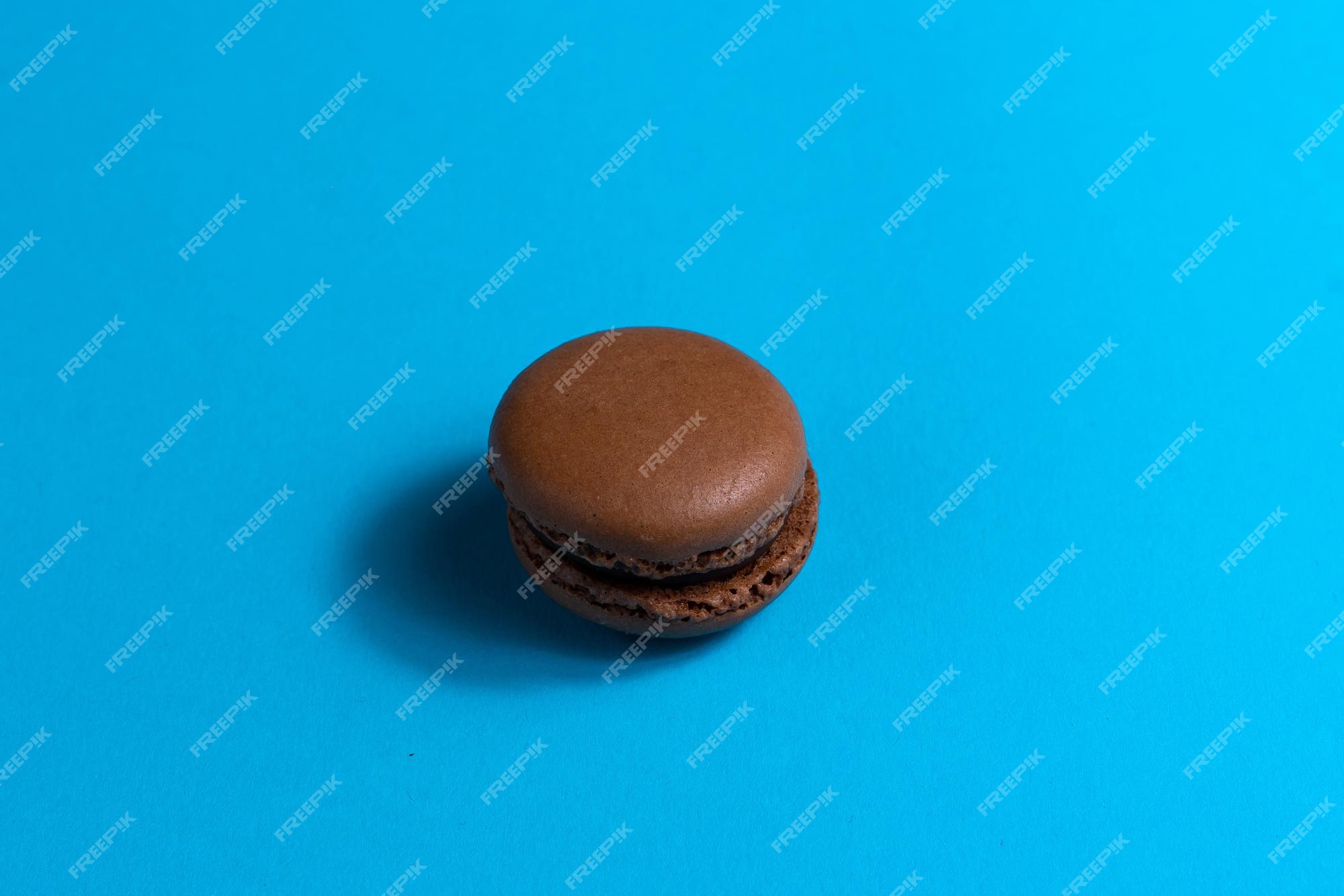The image is a rectangular photograph, approximately six inches wide and three to four inches high, featuring a light blue, textured background that appears darker and more saturated on the left, gradually lightening on the right due to a light source. Centrally positioned is a single, medium to dark brown macaron, likely chocolate-flavored. The macaron comprises two circular pastry halves with a creamy filling; however, the top half is slightly misaligned towards the upper left, revealing a portion of the lower half's edge on the lower right. The macaron casts a bluish-gray shadow to the left. Diagonally across the entire image, from the lower left to the upper right, is a repeating watermark in light blue or gray text that reads "freepik."